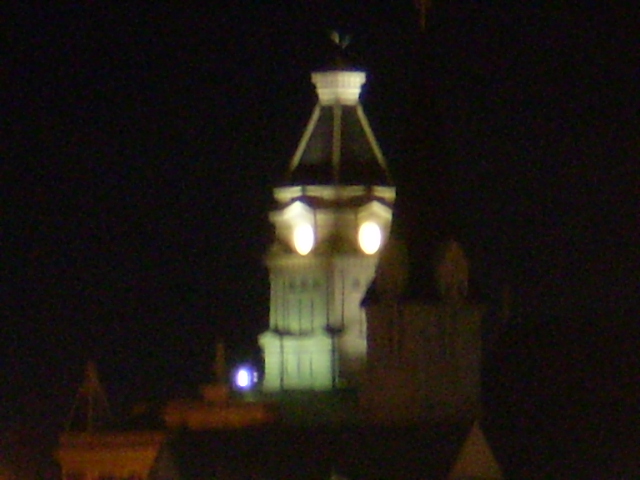The photograph, taken at night, captures an old architectural building, likely a church, with a blurred quality that makes details hard to discern. The primary structure is prominently lit and features a white façade with a triangular, black-colored dome or steeple. In addition to the primary structure, a darkened, similar type of building is visible in the foreground, suggesting the photo was taken from an elevated position. The scene includes white, black, and purple hues, with the purple light shining just beside the illuminated building. Additional amber or orange glows, possibly from street lamps, highlight the lower portions of the white church, contributing to the eerie atmosphere of the nighttime scene.